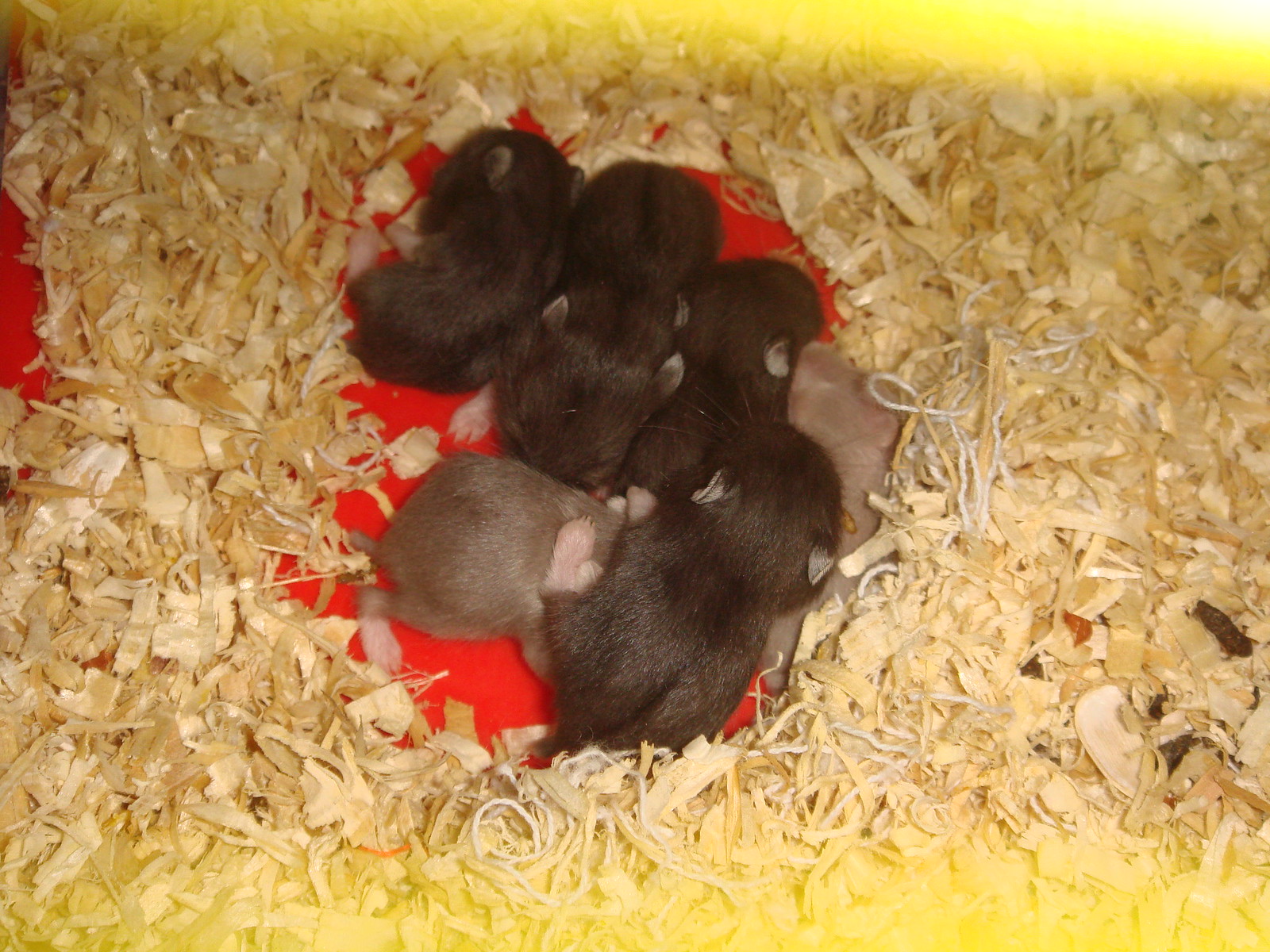This photograph features a close-up of six tiny, newborn mammals huddled together in a nest-like setting within what appears to be a rodent enclosure. These animals, possibly baby hamsters or mice, are nestled on a bright red surface, which is surrounded by a bed of light beige pine shavings. Four of the babies exhibit a dark brown, almost sable coat, while the remaining two display lighter hues of brown. The image is taken from above, capturing the top of their heads and their sleek, compact bodies with stubby tails and tiny ears. The animals are tightly packed, appearing as a single group in the center of the frame. The enclosure features a distinct yellow stripe along both the top and bottom edges. Additionally, there is a faint white string partially buried within the pine shavings. The precise baby animal species remains uncertain, but their healthy, glossy coats and clustered form evoke a sense of warmth and care.